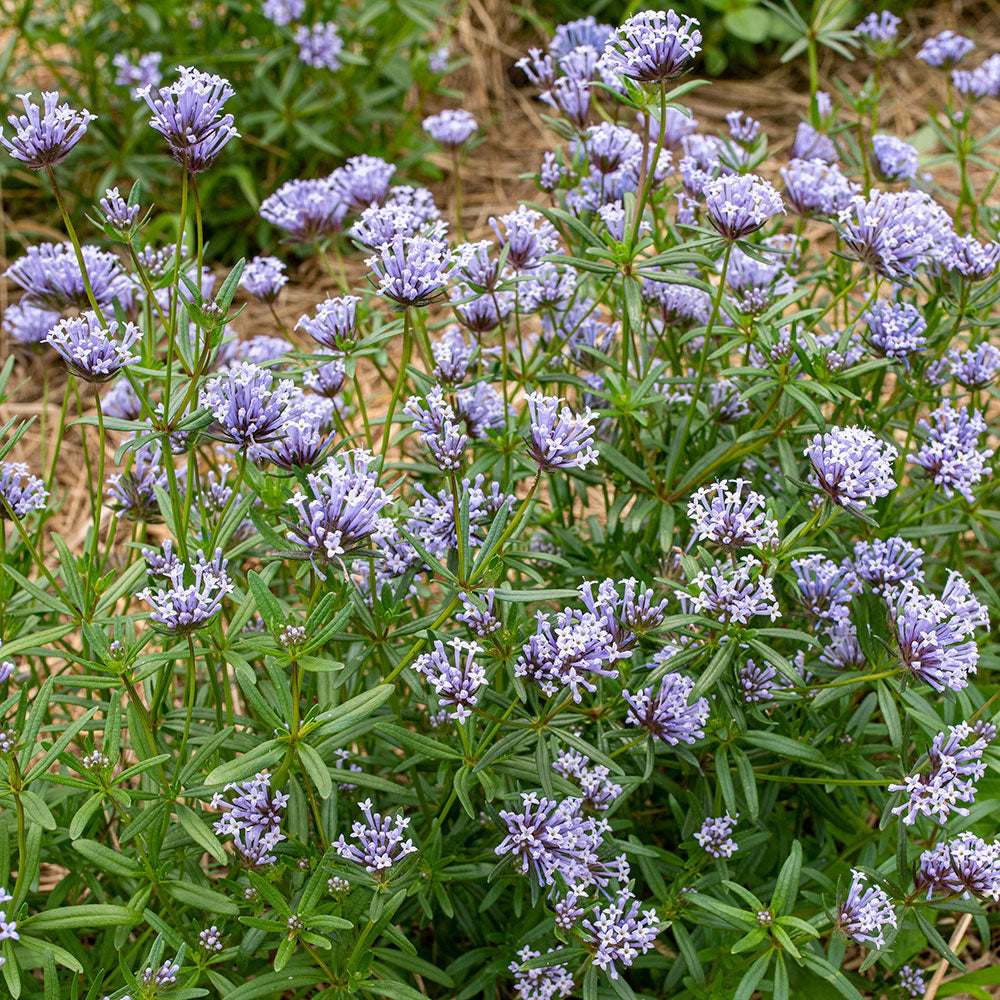The image depicts a close-up scene of numerous small, delicate purple flowers blanketing the ground, bathed in daylight. The flowers are a mix of soft lilac and bluish-lavender hues, with each tiny bloom forming clusters that give the impression of a larger composite flower. The flowers grow on slender green stems, accompanied by elongated green leaves. Beneath and around the flowers, patches of dead or brown grass create a contrast with the vibrant blossoms. The setting appears natural and untouched, with the flowers seemingly flourishing wildly amidst the sparse, dried grass. The focus is entirely on the ground-level flora, with no sky or additional elements visible, emphasizing the organic beauty of these intricate flowers thriving in a modest, untamed patch of earth.